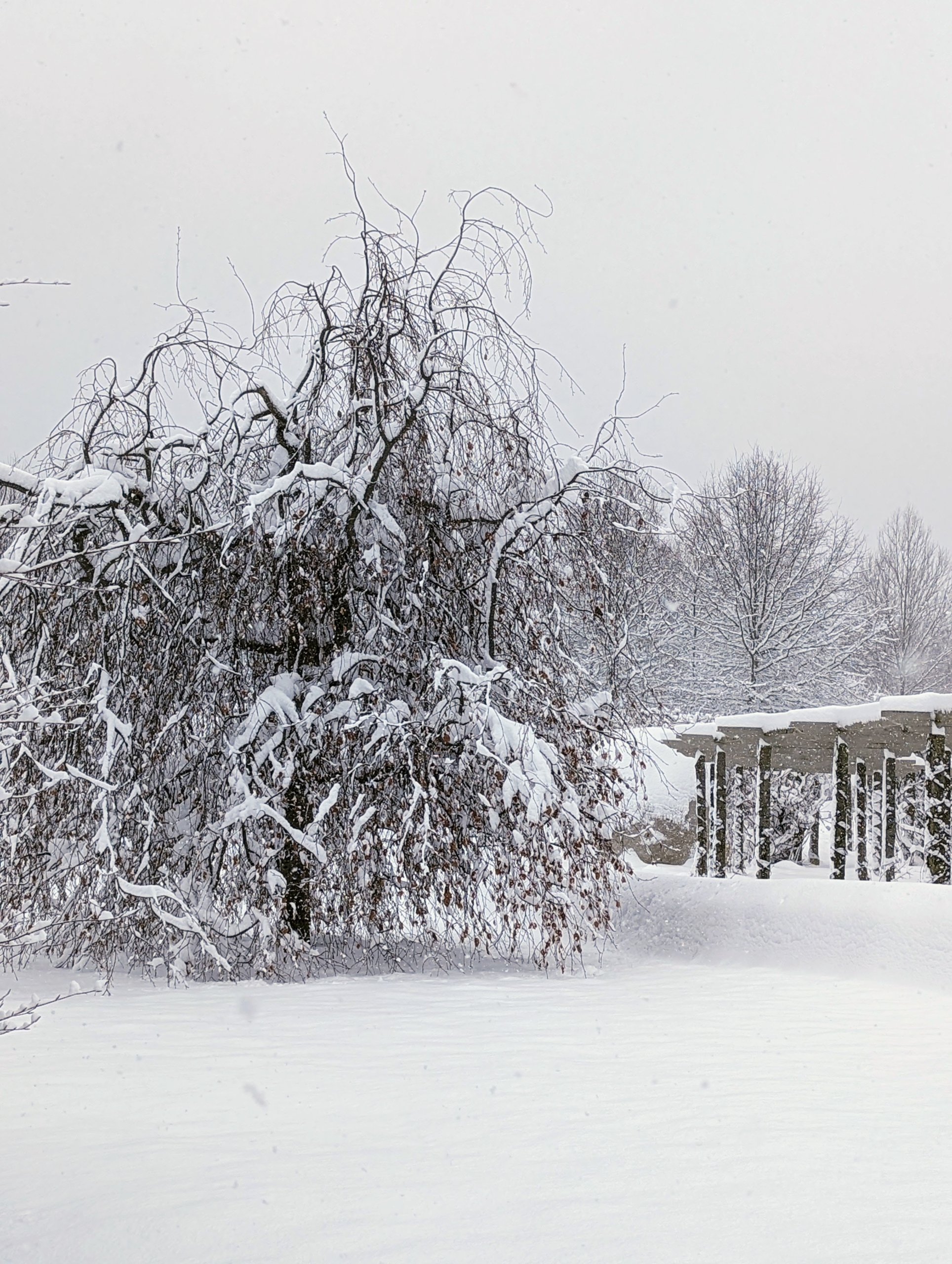The black and white photograph captures a serene winter scene, tall and narrow in orientation. Prominent slightly left of center stands a large tree, potentially a willow, exhibiting twisted, drooping branches heavily laden with snow. The tree’s dark trunk is visible, with its fine twigs reaching skyward, providing a stark contrast to the snow-covered ground beneath. To the right, a structure with multiple dark pillars supports a flat, snow-covered roof, suggesting it might be a carport or porch. The backdrop features several bare-branched trees, possibly elms, oaks, or maples, all contributing to the wintery atmosphere with the ground deeply blanketed in snow. The sky appears as a whitish-gray, completing the monochromatic, snowy landscape.